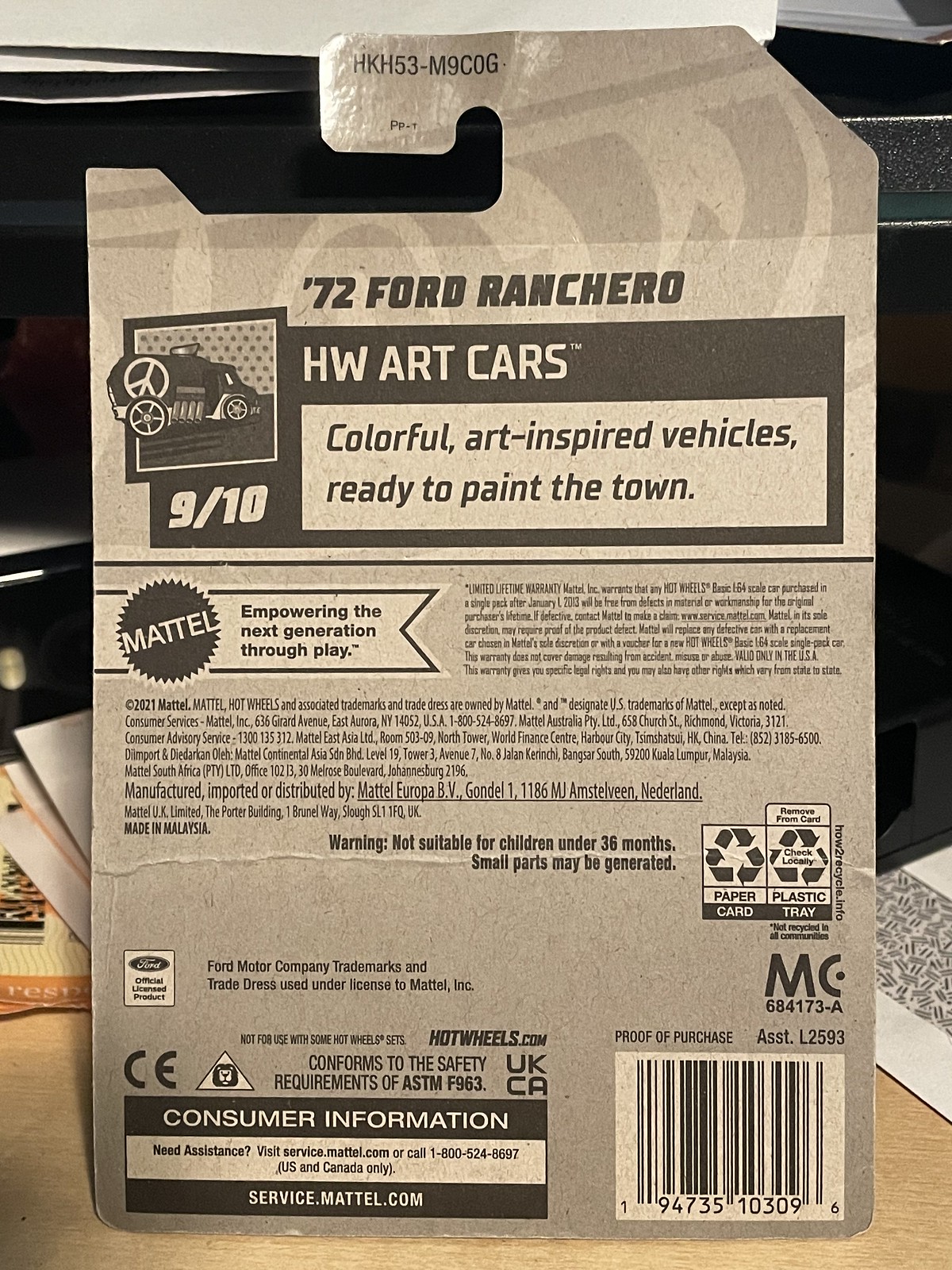The image depicts the back of a cardboard backing for a Hot Wheels toy car. The product is identified as a 1972 Ford Ranchero from the HW Art Cars series, one of the "9 out of 10 colorful art-inspired vehicles ready to paint the town." The back features a small drawing of the vehicle with a peace sign and multiple exhaust pipes. Prominently displayed is the text "Mattel, empowering the next generation through play," alongside the Mattel logo. Additional details include a barcode and proof of purchase number 19473510309 in the bottom right corner, along with fine print that is illegible due to its small size. The packaging also includes a warning: "Not suitable for children under 36 months, small parts may be generated," and notes that the paper card and plastic tray are recyclable. The background appears to be a light beige table, scattered with small pieces of paper and envelopes.